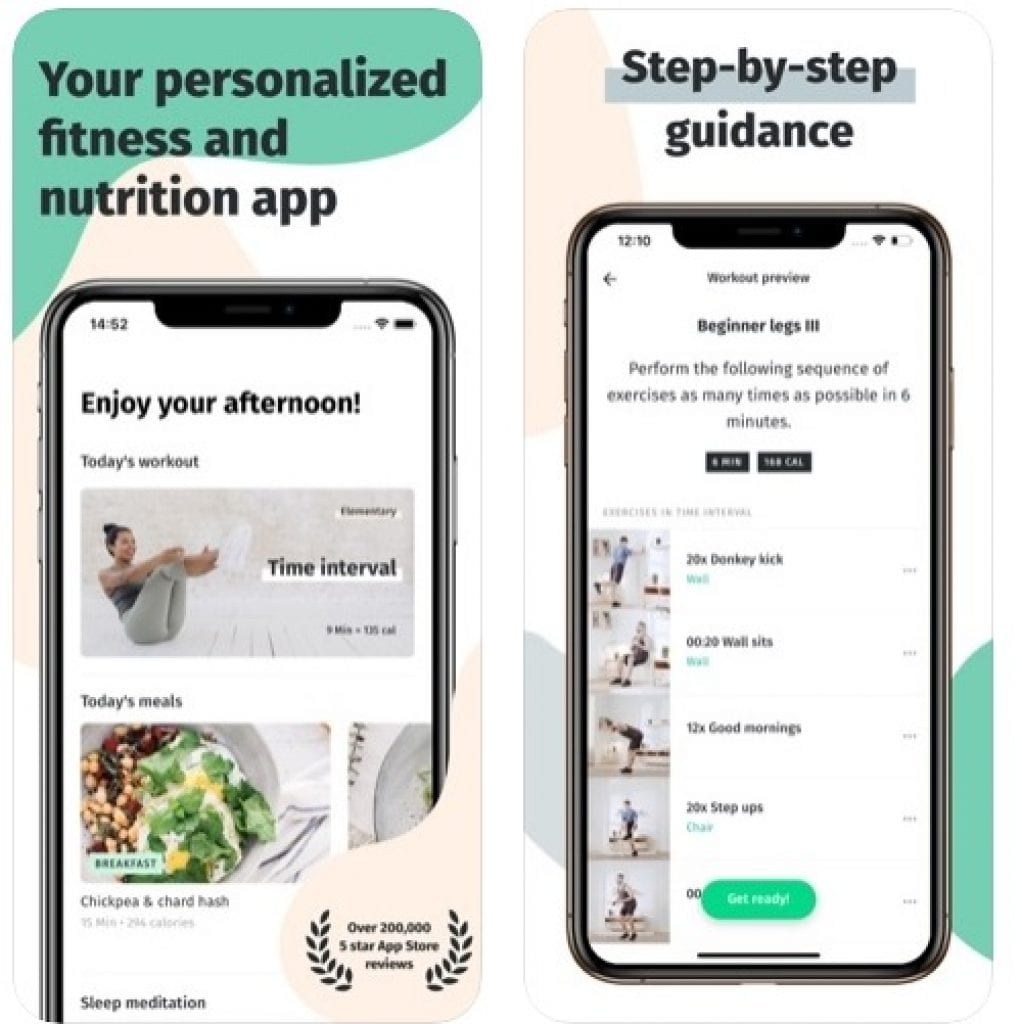In this vibrant promotional image, two iPhones are prominently displayed, each showcasing different features of a fitness and nutrition app. 

The larger background is a blend of calming green at the top, with swirls of peach, white, and gray creating an inviting and dynamic aesthetic. The overarching text reads, "Your personalized fitness and nutrition app," setting the tone for an individualized user experience.

On the first iPhone screen, the app welcomes the user with a message: "Enjoy your afternoon." Below this, it outlines "Today's Workout" along with a specific time interval, featuring a motivational image of a woman in mid-exercise. The meal section highlights a delicious dish with a high-quality image of "Chickpea and Charred Hash." The wellness features of the app include "Sleep Meditation," and the impressive user satisfaction is boasted with "Over 200,000 five-star App Store reviews."

The second iPhone screen provides a detailed "Step by Step Guidance" for a beginner's leg workout. It offers a "Workout Preview" and instructions to "perform the following sequence of exercises as many times as possible in six minutes." An illustrative diagram guides users through exercises such as donkey kicks, wall sits, 'Good Mornings,' and step-ups. A green bar saying "Get Ready" obscures part of the final exercise, followed by a black bar creating a clear separation.

Overall, the image's cohesive background of green, peach, white, and gray enhances the app's modern and user-friendly design, making fitness and nutrition approachable and personalized.